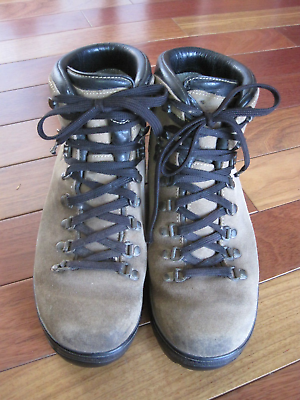In this detailed photograph, a pair of hiking boots are carefully placed together, touching slightly. Each boot is crafted from light brown buffed leather with a small black scuff on the very front of the toes. The boots feature black soles and thick black laces tied neatly at the top. The lacing eyelets appear to be gold, adding a touch of contrast. Around the top, there is cushioned black leather for added comfort, and this continues onto the top part of the tongue of the boots. The tongues themselves are primarily a suede brown, matching the main material of the boots. The hardwood floor that serves as the backdrop for the boots is composed of rectangular planks in varying shades of brown, ranging from light tan to darker hues, with a noticeable shine reflecting light at the top of the image. The boots are centrally positioned, creating a balanced and composed scene.